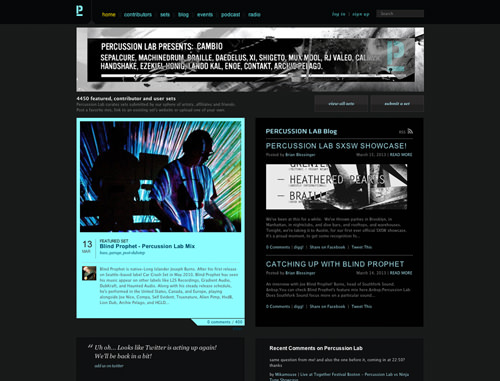The image consists of various rectangular shapes and different sections filled with diverse texts and graphics primarily in blue, gray, black, and white tones, arranged in a structured format.

The top section features a black rectangle, followed by a dark gray rectangle immediately underneath it. Prominently at the top, there is a blue-colored "P" with an accompanying word beneath it. 

Below this, a gold-colored word is followed by more blue text aligned to the right. In the central section, there is a black-and-white picture, partially obscured by a gray, semi-transparent overlay rectangle, featuring white text and underscored by a white line.

To the left side, another blue "P" appears with text beneath it. This is succeeded by additional white text followed by gray text. The right side features blue text enclosed within small gray rectangles.

Further down, a notable blue rectangle with a tab at the bottom contains an image of a person silhouetted against another figure, possibly involving a computer screen, and several lines. Text indicating "13" along with another word is followed by a line and additional words to the right of it. A small, indiscernible square picture is included here, with more text alongside.

The tab contains more words, and just beneath this section, within a black rectangle, there are white words. On the right-hand side, another black rectangle contains light blue text. There’s also a black-and-white picture with overlaid writing, which is not clear, accompanied by additional gray text. Beneath this appears blue text separated by a thin gray line.

Towards the bottom, the phrase "Catching Up with Blind Prophet" is prominently displayed in blue text. Following this heading, more white and gray text is visible. Finally, a gray rectangle with white and gray writing concludes the descriptive contents of the image.